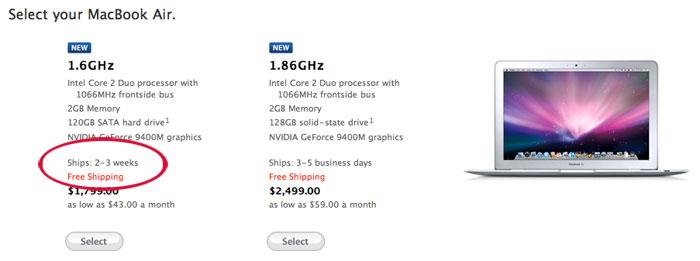In the image, a webpage featuring two models of MacBook Air laptops is displayed against a white background. The left side of the page is divided into two sections, each detailing a different laptop model.

At the top of the left section, the text "Select your MacBook Air" is prominently displayed in black. Below, the first model is introduced with a blue button labeled "New" in white text, indicating the model features a 1.6 GHz Intel Core 2 Duo processor. The details provided in the description include: 
- Intel Core 2 Duo processor with a 1066 MHz front-side bus
- 2 GB of memory
- 120 GB SATA hard drive
- NVIDIA GeForce 9400M graphics

Highlighting the shipment details, a red circle emphasizes "Ships: 2-3 weeks, free shipping." The price is listed at $1,799 with financing options as low as $43 per month. A gray "Select" button is included below the price.

The second model, positioned beneath the first, features a 1.8 GHz Intel Core Duo processor with similar attributes but with a 128 GB solid-state drive. Shipping details mention "Ships: 3-5 business days, free shipping." This model is priced at $2,499 with financing options starting at $59 per month, accompanied by a similar gray "Select" button.

On the right side of the image, a picture of the MacBook Air is displayed against a space-themed background. The laptop appears in a sleek silver finish, accentuating its aesthetic appeal.